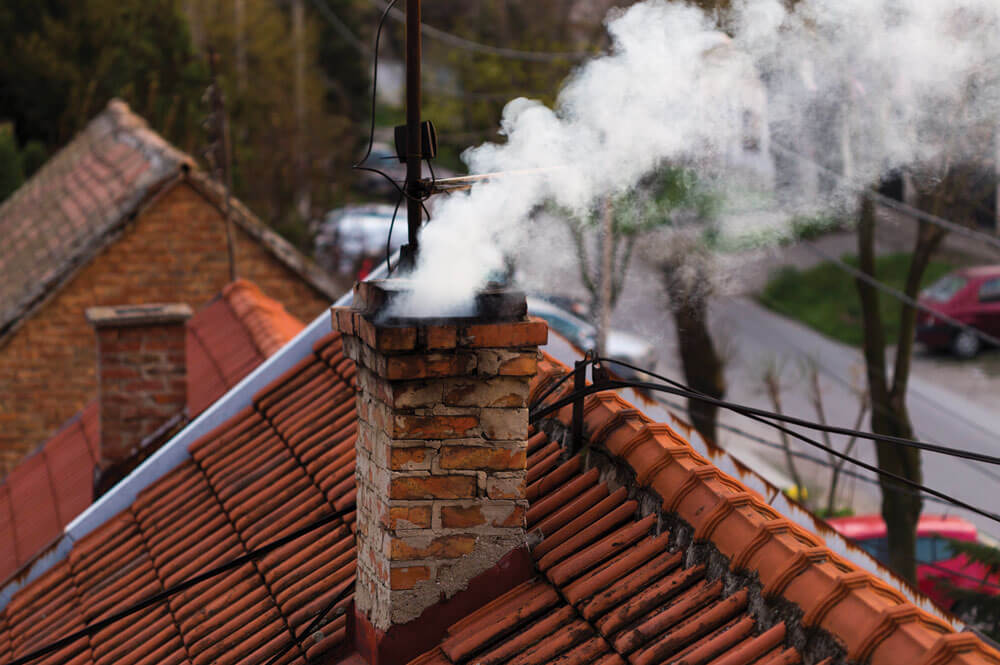The image captures an outdoor scene featuring a red terracotta or shingle roof with two brick chimneys. The primary focus is on the main chimney, which stands robustly in the center of the frame, emitting a plume of white smoke that drifts to the top right of the image. This chimney appears weathered and has multiple black wires—likely power or phone lines—attached to it and the roof. In the background, stretching to the left, sits another roof with a secondary chimney that shows no signs of smoke. The background also reveals a bustling street with a mix of red and white cars, bordered by bare trees indicative of fall or winter. A notable red vehicle is parked at the bottom right corner between two trees, near the edge of the rusty metal roof line. Despite the cloudiness of the sky, the entire setting gives a glimpse into a quaint, slightly aged neighborhood landscape.